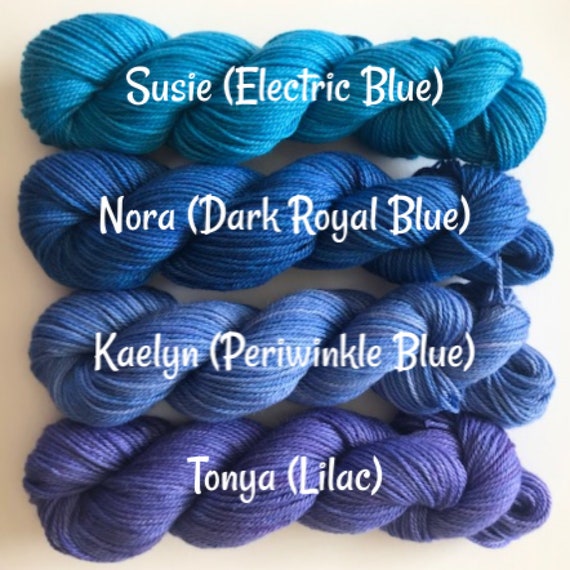This photograph features four horizontally aligned skeins of yarn, each meticulously twisted into long bundles and placed on a yellowish-white surface. The skeins, varying in shades of blue and purple, display white text labels with women's names and specific color descriptors, positioned from top to bottom. The first skein is labeled "Suzy" with the color "Electric Blue," a light turquoise shade. The second skein, "Nora," is "Dark Royal Blue," a deeper, rich blue. Third in line is "Kaelin," described as "Periwinkle Blue," a blend of light and even lighter blue hues. The final skein, "Tanya," is "Lilac," presenting a soft light purple color. Each bundle is twisted into a two-strand twist, with ends neatly tucked inside, showcasing no loose strands. The background and text coordinate in white, emphasizing the vibrant colors of the yarn.